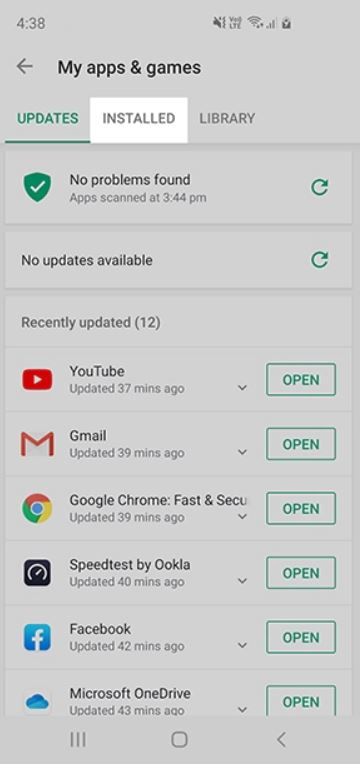**Detailed Caption:**

The screenshot is from an Android phone displaying the "My Apps & Games" section in the Google Play Store. The time shown at the top left is 4:38 PM, accompanied by icons indicating LTE, Wi-Fi, and mobile cellular signals.

Below the status bar, the navigation header reads "My Apps & Games" with a back button on its left. The background predominantly features a light gray shade. The interface is divided into three tabs: "Updates," "Installed," and "Library," with the "Installed" tab highlighted by a whitish rectangle.

Directly underneath, there's a message that reads "No problems found," accompanied by a green shield icon with a checkmark in the center. Below this, it states "Apps scanned at 3:44 PM" with a refresh button to the right.

Further down, it indicates "No updates available," again with a refresh button beside this message.

Following that, the section labeled "Recently updated (12)" appears. The list includes:

1. **YouTube** - Updated 37 minutes ago, with a green "Open" button to the right.
2. **Gmail** - Updated 39 minutes ago, with an "Open" button to the right.
3. **Google Chrome: Fast & Secure** - Updated 39 minutes ago, also with an "Open" button on the right.
4. **Speedtest by Ookla** - Updated 40 minutes ago, with an "Open" button to the right.
5. **Facebook** - Updated 42 minutes ago, followed by an "Open" button.
6. **Microsoft OneDrive** - Updated 43 minutes ago, accompanied by an "Open" button on its right.